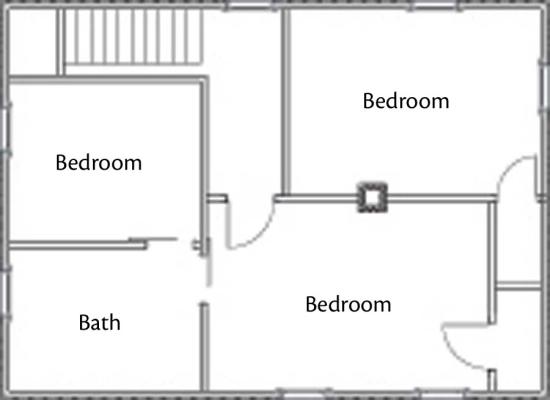This architectural blueprint highlights the layout of a second-story floor plan, featuring three bedrooms and a bathroom. The double black line outline signifies the perimeters of the area. 

Starting at the upper left-hand corner, there is a small landing connected to a staircase heading right. The stairs lead to a hallway, enclosed by walls on both sides, where you would need to make a right turn at the top. Directly ahead at the end of this hallway is a bedroom, accessible through a door that opens inward to the right. Inside this bedroom, a short wall houses a pocket door that slides into a bathroom located in the left corner.

Within the bathroom, taking a sharp right after the pocket door leads to another pocket door, which opens into the adjacent bedroom next to the stairs, forming part of the hallway wall. This setup allows both the bedroom and the bathroom to be interconnected via pocket doors.

The third bedroom is notably spacious. In the bottom right corner, there’s a door that opens into the room and provides access to a closet area. However, there appears to be no direct entry into what seems to be a fourth bedroom situated in the upper right-hand corner of the drawing. Instead, to reach this additional space, one would have to navigate through the third bedroom, moving along its right side into a narrow closet that runs alongside another closet designated for the bedroom at the end of the hallway.

Notably, there is a square, darkened area positioned between the two bedrooms, possibly an access point to the attic or another utility space.

In summary, this blueprint reveals an intricate design with interconnected rooms, featuring pocket doors for efficient use of space but lacks clear access to the potential fourth bedroom.